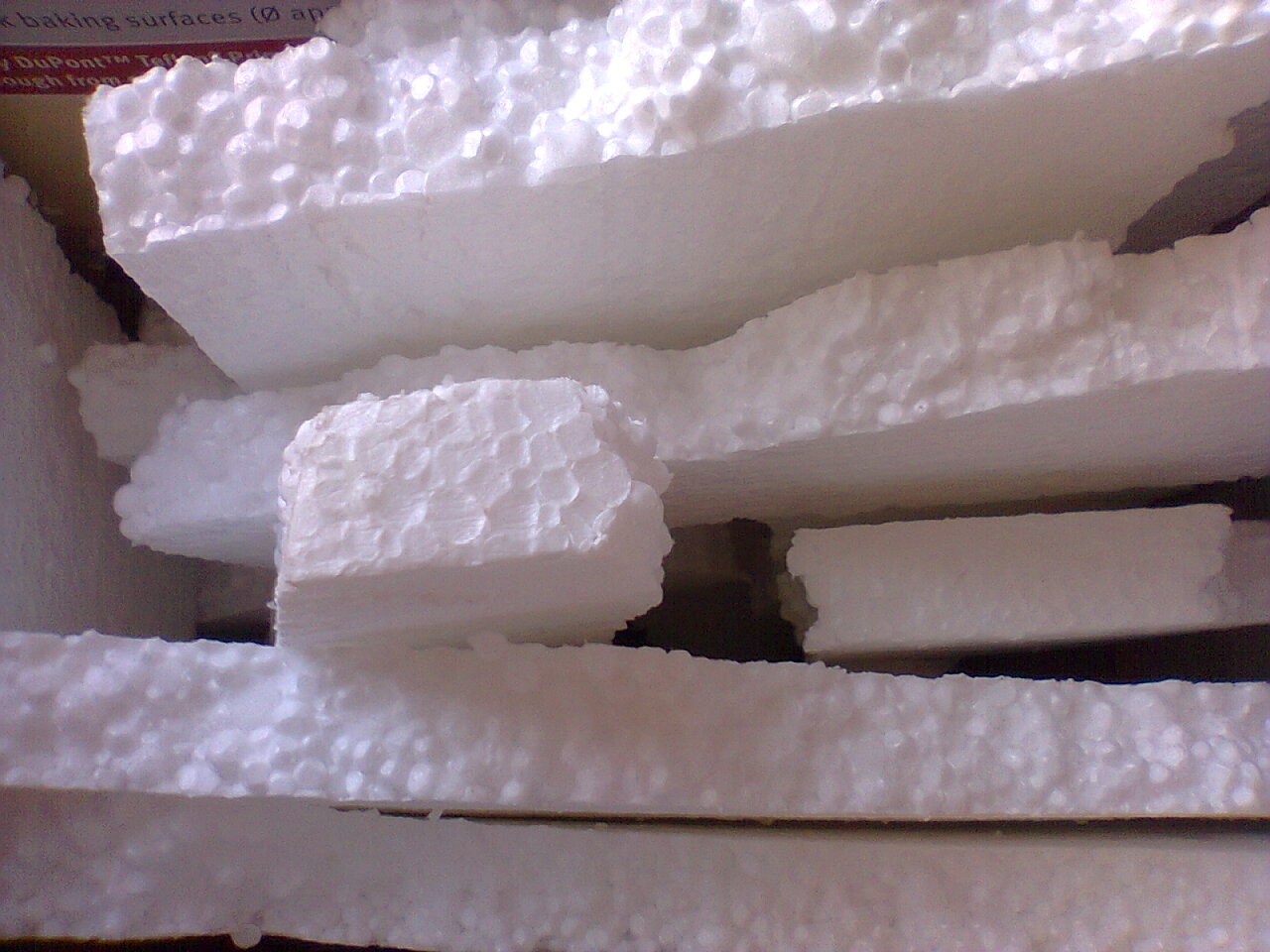This image features seven pieces of bright white Styrofoam, each with jagged, ripped edges. The Styrofoam pieces are stacked vertically on their sides, creating a somewhat organized yet haphazard arrangement, with the jagged edges facing upwards. The pieces are nestled closely together, forming noticeable gaps between them in certain areas, particularly toward the middle of the image. In the upper-right corner, there is text in black lettering that reads "baking surfaces." Below this text is a red strip with white lettering that includes the DuPont trademark and partial text "Teflon something." This suggests the Styrofoam might have been part of packaging material. The image is devoid of any identifiable information, such as a date, location, or people, and is possibly taken inside a box.